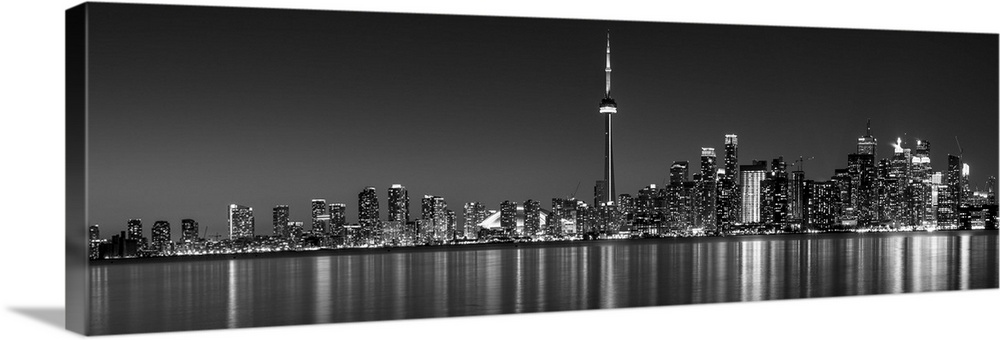In this detailed black and white panoramic image, we see the majestically lit nighttime skyline of a bustling city, reminiscent of iconic American metropolises like New York, Chicago, or even Seattle. Dominating the canvas is a dramatic array of tall skyscrapers, particularly concentrated on the right side, with a singular, prominent tower standing proudly near the center. To the left, the buildings gradually decrease in height, providing a balanced yet dynamic cityscape. The skyline forms a striking contrast against the unyielding, dark gray sky, free from cloud cover. Below, a serene body of water stretches across the bottom of the image, capturing the luminous reflections of the city lights. Viewing the image from a slightly front diagonal perspective, the entire scene is presented within a rectangular canvas, with the physical edges of the picture frame visible to the left. The art itself rests in a minimalistic setting that suggests it could be a high-quality, displayed photograph, perhaps intended for sale or advertisement. The overall composition, highlighted by deep shadows and brilliant reflections, beautifully encapsulates the essence and vibrancy of an urban nocturnal landscape.